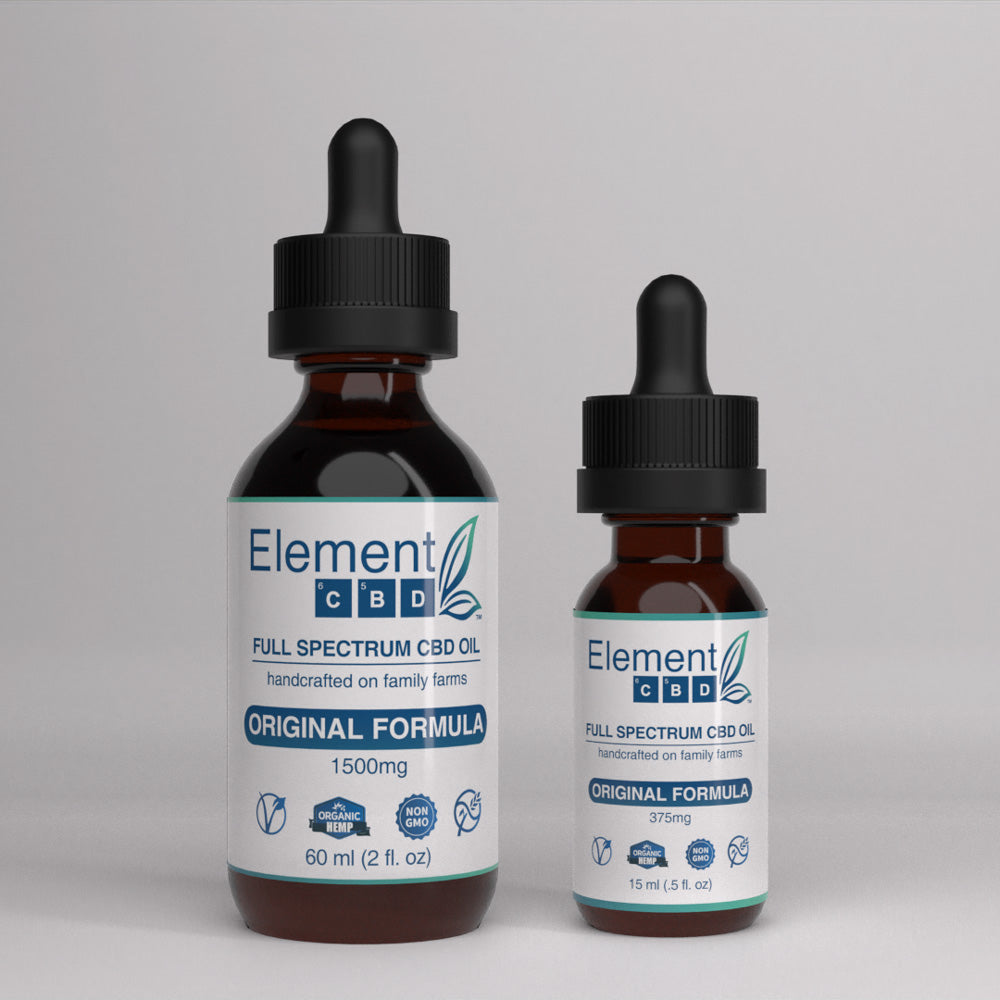The image depicts two dark amber glass bottles with dropper tops, positioned side by side on a greyish surface with a grey background. Both bottles are identical in design, featuring black rubber caps with droppers. The larger bottle on the left has a capacity of 60 milliliters (2 fluid ounces) and contains 1500 milligrams of Element CBD full-spectrum CBD oil, while the smaller bottle on the right holds 15 milliliters (375 milligrams). Each bottle has a white label with blue lettering that reads "Element CBD," along with green and blue leaf logos. The label also states "Full Spectrum CBD Oil, Handcrafted on Family Farms, Original Formula," and includes additional blue and white symbols for organic hemp and non-GMO certifications.